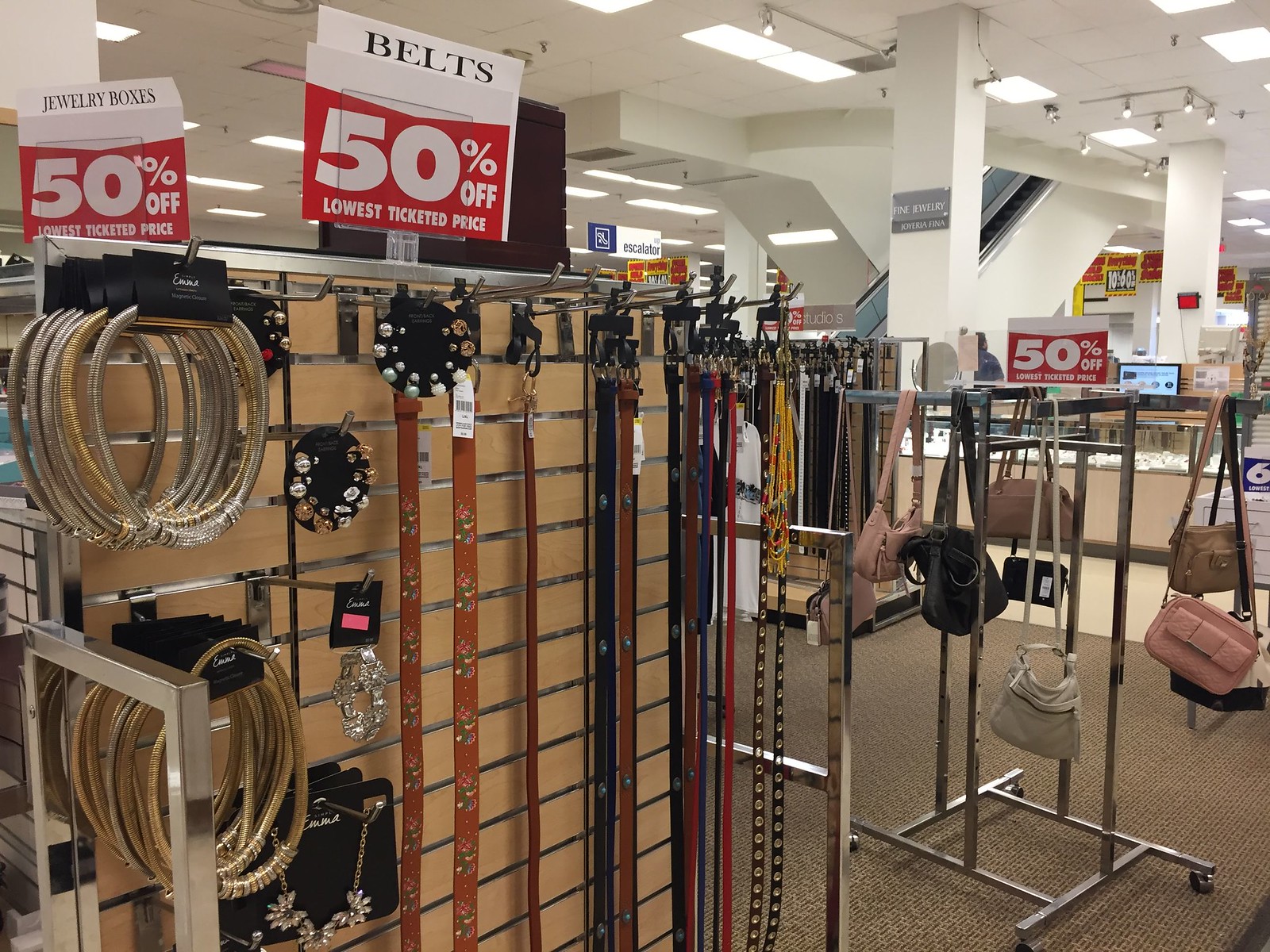This image depicts the accessory section within a bustling department store. The foreground showcases a large, organized rack filled with various belts, presenting an assortment of styles and colors. Adjacent to the belts, an eye-catching selection of jewelry, including bracelets and necklaces, is delicately displayed. To the right of this assortment, a separate rack features an array of purses, each carefully hung for easy browsing. Overhead, a prominent sign boldly announces a 50% off discount on the lowest ticketed prices, printed in white against a vibrant red background. The upper portion of the image reveals structural details of the store, including pillars, the ceiling, and a visible escalator, hinting at the expansive layout. The section is grounded by a brown carpet, providing a warm contrast to the glimmering accessories and enhancing the shopping experience.